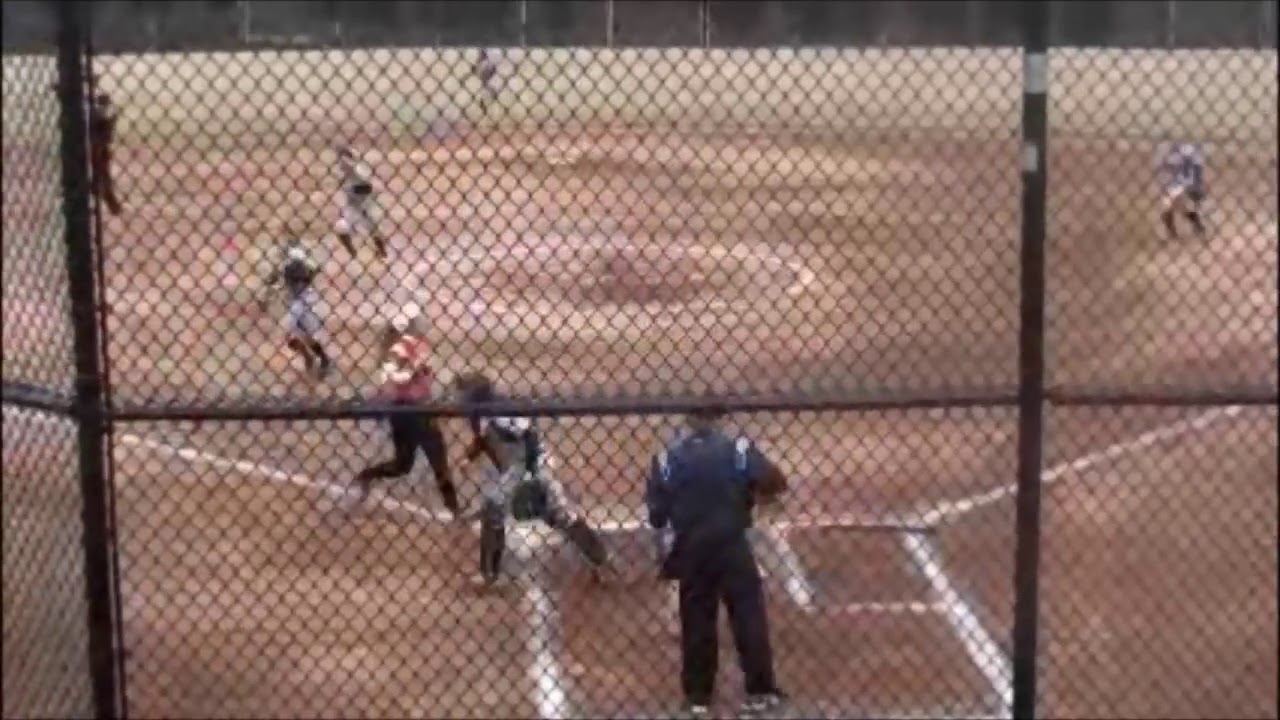In this dynamic and slightly blurry horizontal photograph, a spirited girls' softball game is captured from behind a tall, black chain-link fence. The picture shows a dirt field meticulously marked with white outlines, including home plate and the large circle at the pitcher's position, confirming it's a softball game. Central to the scene is an umpire clad in blue, standing behind the batter's box and looking out onto the field. 

In the foreground, a catcher wearing a white uniform is moving to the left outside the batter's box, possibly preparing to intercept the play. A thrilling moment is frozen in time as a runner donning an orange top, black pants, and a distinctive white helmet sprints down the third baseline, aiming for home plate. Meanwhile, the fielders, dressed in gray jerseys with black socks, are seen heading off the field, likely having just secured the third out. The defensive team includes five visible players scattered across the infield and outfield, including one stationed near first base in a blue top and another visible in the distant outfield where the grass turns a lush green.

The rich details of the players’ movements, their vibrant uniforms, and the structured environment all contribute to the sense of excitement and teamwork characteristic of a lively little league softball game.